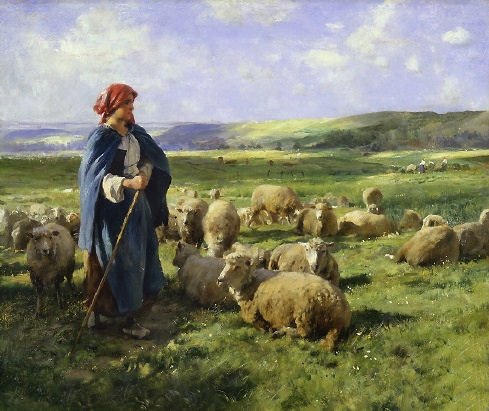The painting depicts a serene outdoor scene during the day, featuring a shepherd, likely a woman, in a lush green field dotted with sheep. The shepherd is holding a long, brown staff with her right hand and is dressed in a combination of robes. She wears a white upper garment, a blue and brown skirt, and a red scarf covering her head. The sheep, varying in posture with some standing and others lying down, have dark gray bodies with lighter gray heads. In the background, rolling hills give way to towering, green-covered mountains. The sky is a vivid blue, speckled with puffy and wispy white clouds. The shepherd gazes thoughtfully into the distance, adding a contemplative mood to the idyllic landscape.